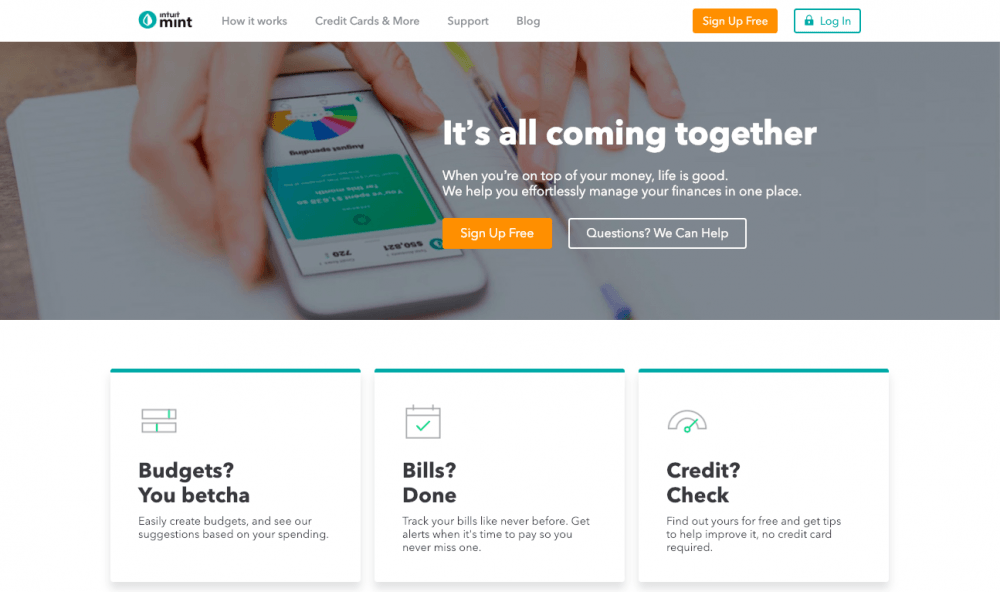The image is a screenshot of the homepage of the Intuit Mint website. At the top left corner, the name "Intuit Mint" is prominently displayed. The navigation menu includes sections titled "How It Works," "Credit Cards," "More," "Support," and "Blog." 

In the central area of the homepage, a significant headline reads, "It's all coming together. When you're on top of your money, life is good. We help you effortlessly manage your finances in one place." Below this welcoming message, there is a call-to-action button labeled "Sign Up Free." To the lower right of this button, another button reads, "Questions? We can help."

Further down, the homepage features three cards with individual titles and descriptions. The first card, titled "Budgets You Betcha," explains, "Easily create budgets and see our suggestions based on your spending." The second card, "Bills? Done," elaborates, "Track your bills like never before. Get alerts when it's time to pay so you never miss one." The third card, titled "Credit? Check," states, "Find out yours for free and get tips to help improve it. No credit card required."